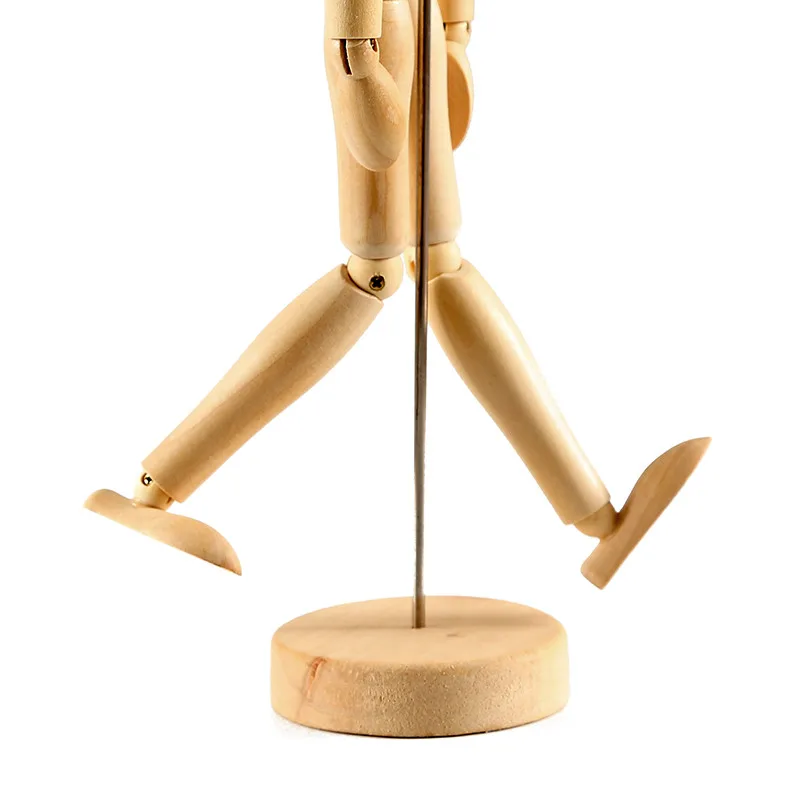The image shows the lower half of an undressed wooden puppet displayed on a round, beige-colored wooden base. A slender black metal rod extends vertically from the base, supporting the puppet. The visible parts of the puppet include jointed legs that are positioned as if in the motion of walking, with one foot stepping forward while the other is drawn back. The legs are connected to soft, rounded thigh sections that join at flexible knee and ankle joints. The puppet’s feet have swivels, and its hands are shaped like paddles without distinct fingers. The screws at the joints of the knees, wrists, and ankles are visible. The upper body of the puppet is cut off from the image, leaving only the detailed view of its lower portion against a white background.